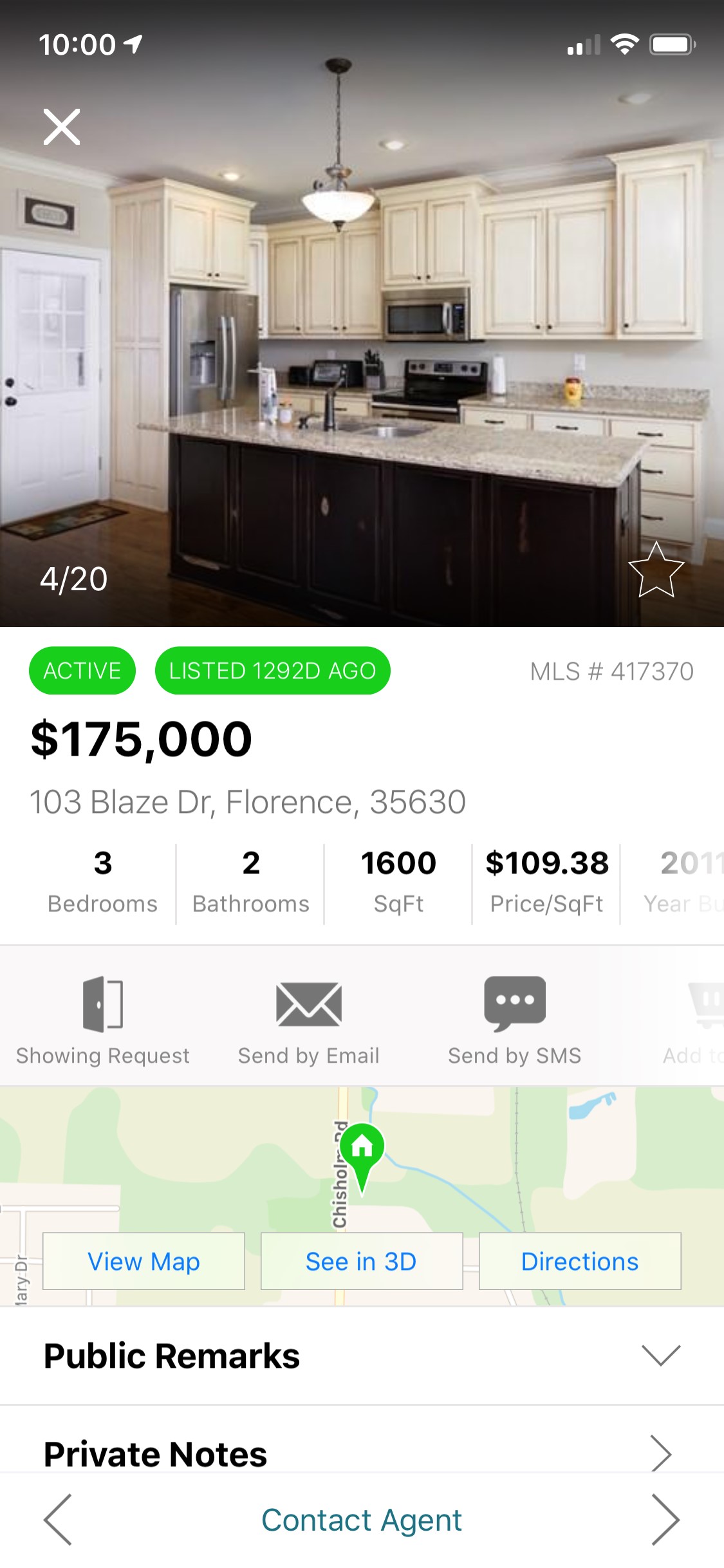In this image, a user is browsing home listings for an apartment located at 103 Blaze Drive, Florence, zip code 35630. The focal point of the image is the fourth of 20 photos, showcasing a stunning, modern kitchen. Above the image, green text indicates that the listing has been active for 1,292 days. The apartment is priced at $175,000 and offers three bathrooms and two bedrooms, encompassing a total of 1,600 square feet, which breaks down to $109 per square foot.

Beneath the listing details, a gray task bar provides options to request a showing, send an email, or send an SMS. Just below that, part of the screen displays a map showing the apartment's location, which can be viewed in either 3D or normal mode. Further down, there are sections for public remarks and private notes.

The entire interface is displayed in a monochromatic theme of black and white, making it visually clean and straightforward, except for the green text highlighting the active listing status. The app design is minimalistic, focusing on functionality and ease of viewing.